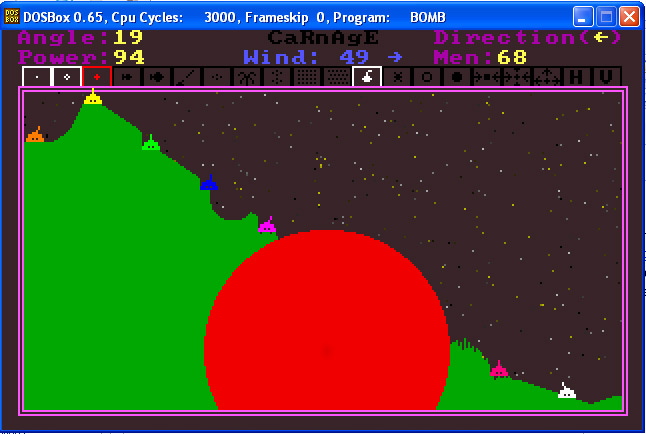This image is a detailed screenshot of an older-style video game, displayed within a DOSBox emulator running on a Windows XP-like interface. The window features the classic bright blue bar at the top labeled "DOSBox 0.65," with white text indicating "CPU Cycles 3000," "Frameskip 0," and the program name "BOMB." The window includes the familiar minimize, grayed-out maximize, and red exit buttons.

The game screen depicts a night sky background with yellow, gray, and white dots representing stars. Central to the image is a pixelated, simplified green hill with numerous small buildings or objects colored in orange, yellow, green, blue, pink, red, and white. Prominently placed in the lower middle part of the screenshot is a red circle overlaying the green area. Additionally, game data scattered around the scene includes text such as "angle 19," "power 94," "wind 49," with an arrow pointing to the left, and "men 68." This detailed setup, combined with the pixelated graphics, indicates the game might be a retro style, tying back to the DOS era of gaming.